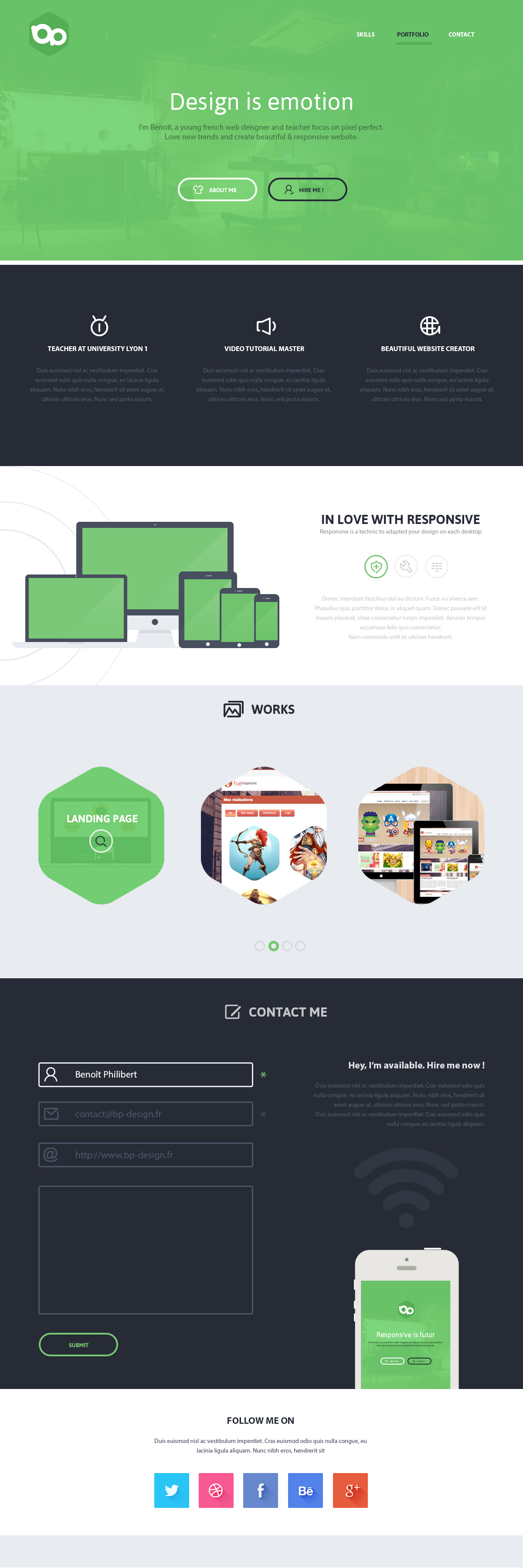A screenshot of a sleek and modern website showcasing a sophisticated design theme in shades of green and black. The primary content area features a white background with multiple embedded images. At the top, a prominent header reads "Design is Emotion," accompanied by navigation options for further exploration. Directly below, a black strip provides an overview of the website’s purpose, illustrated by various images of computer screens representing different types of electronic devices to emphasize the theme of responsive design. An inscription, slightly unclear but suggesting a passion for responsiveness, is partially visible. Following this section, a gallery titled "Works" displays three additional images, likely showcasing more electronic devices or design projects. Finally, at the bottom, a black-labeled "Contact Me" section invites user interaction with fillable information bars. In the lower-right corner, a phone icon with signal strength bars hints at connectivity, though the accompanying text is not entirely readable.